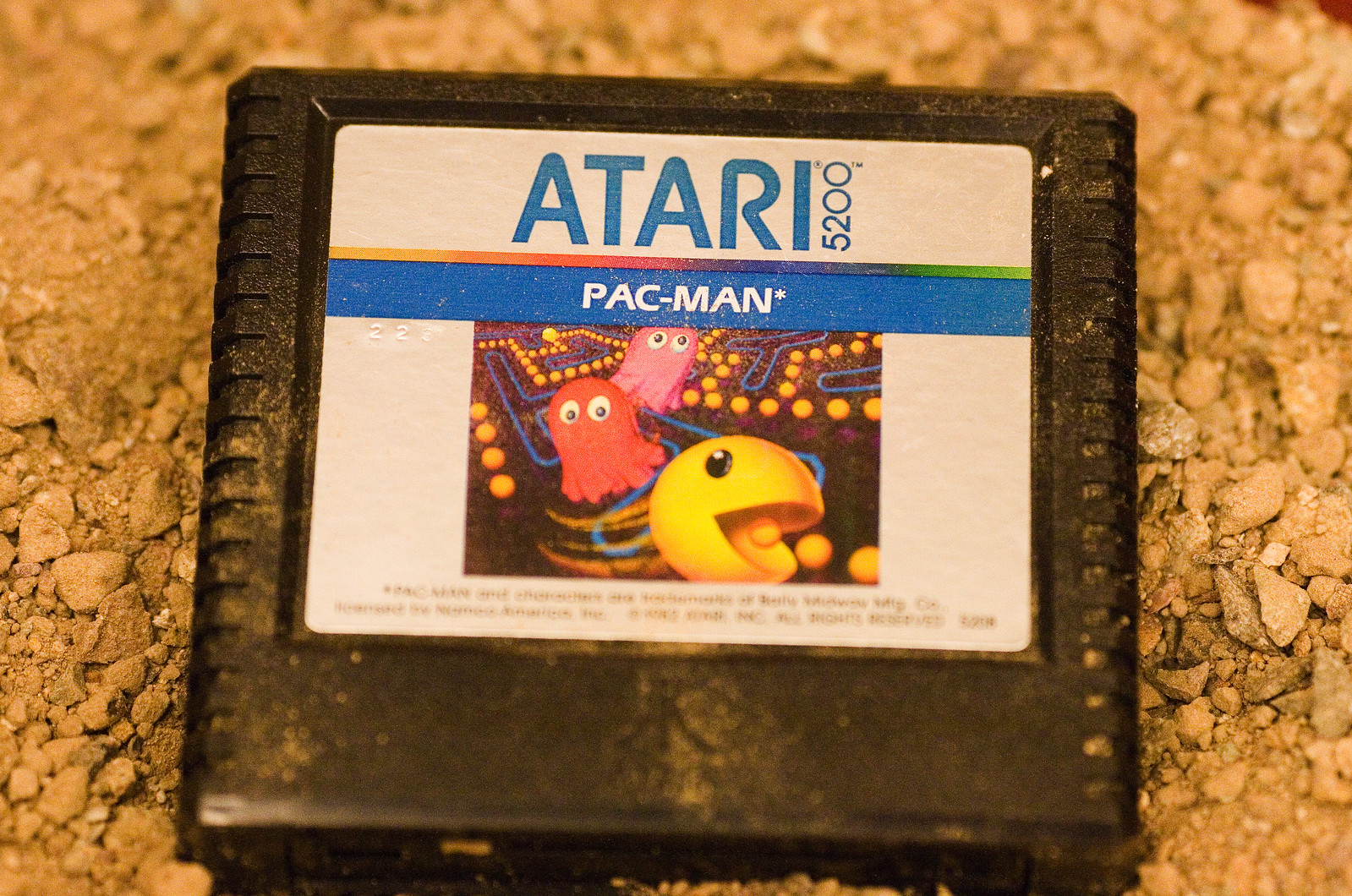This close-up image features a vintage Atari 5200 Pac-Man game cartridge. The cartridge, which is predominantly black, appears aged and coated with a significant layer of dust and grime. The label on the cartridge, although obscured by the debris, showcases a white background with blue Atari branding at the top. The title "Pac-Man" is prominently displayed, accompanied by a stylized illustration of Pac-Man eating pellets and being pursued by red and pink ghosts. The image background suggests an outdoor setting, possibly on rocks or dirt, as the cartridge is surrounded and partially covered by soil, lending to its weathered and neglected appearance.